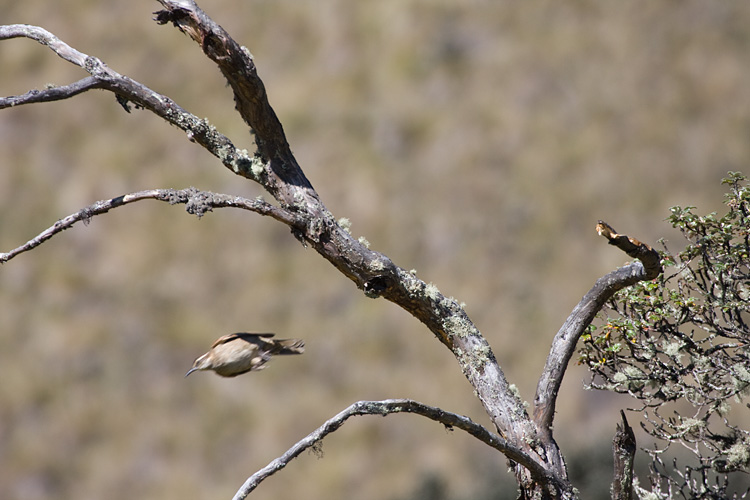In this outdoor photograph, a dead, fungus-eaten branch extends from the bottom center towards the top left of the image. The branch, which is a mix of grayish and brown hues, appears quite aged and possibly diseased. To the left of the branch, a small, stocky brown and white bird, resembling a fat finch, is captured mid-flight, seemingly diving towards the bottom left with its black beak leading the way. Its wings are tucked close, and its overall flight posture suggests a dynamic descent. On the right side of the image, a rotting bush with sparse, gray-green leaves reaches towards the branch. The background is a mix of blurry, muted colors – gray, brown, green, and hints of beige and white – giving a sense of an indistinct, possibly woodland, setting.